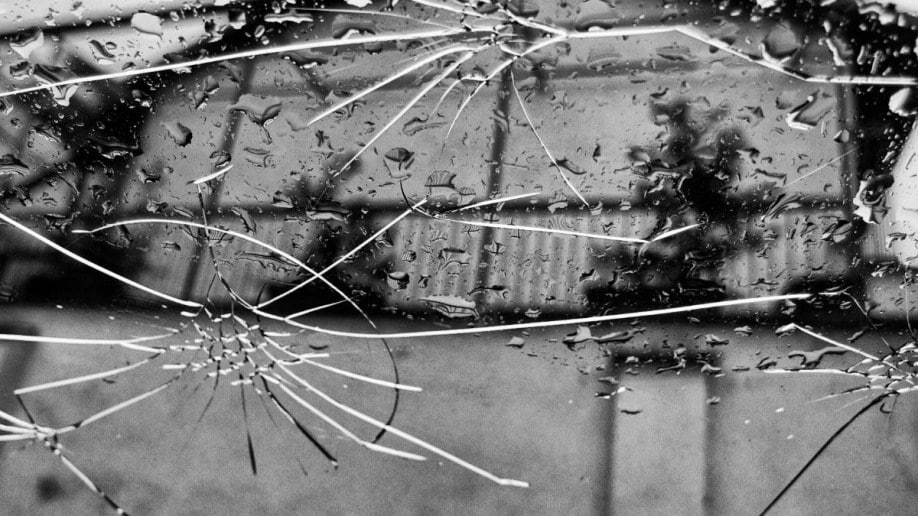This black-and-white photograph captures a close-up view of a pane of glass with extensive spider-webbed cracks, reminiscent of a shattered window. The large, prominent crack stretches like a lightning bolt across the upper portion, intersecting with several smaller fissures that radiate outward, creating a complex and chaotic pattern. Additionally, a pronounced half-circle crack can be noticed at the bottom, along with distinct web-like cracks in the bottom left corner extending toward the right.

Drops of water cling to the surface of the glass, indicating that it has recently rained or is still raining, creating a wet, reflective sheen. Beyond the cracked glass, shadows and outlines depict a building structure, marked by dark lumber frames interspersed with lighter materials. Silhouettes of railings and possibly small trees or bushes in the dreary, gray background add depth and atmosphere, enhancing the melancholic and somber mood of the photo. The ambiguity of whether the glass is a window or a reflective mirror further adds to the intriguing mystery of the scene.